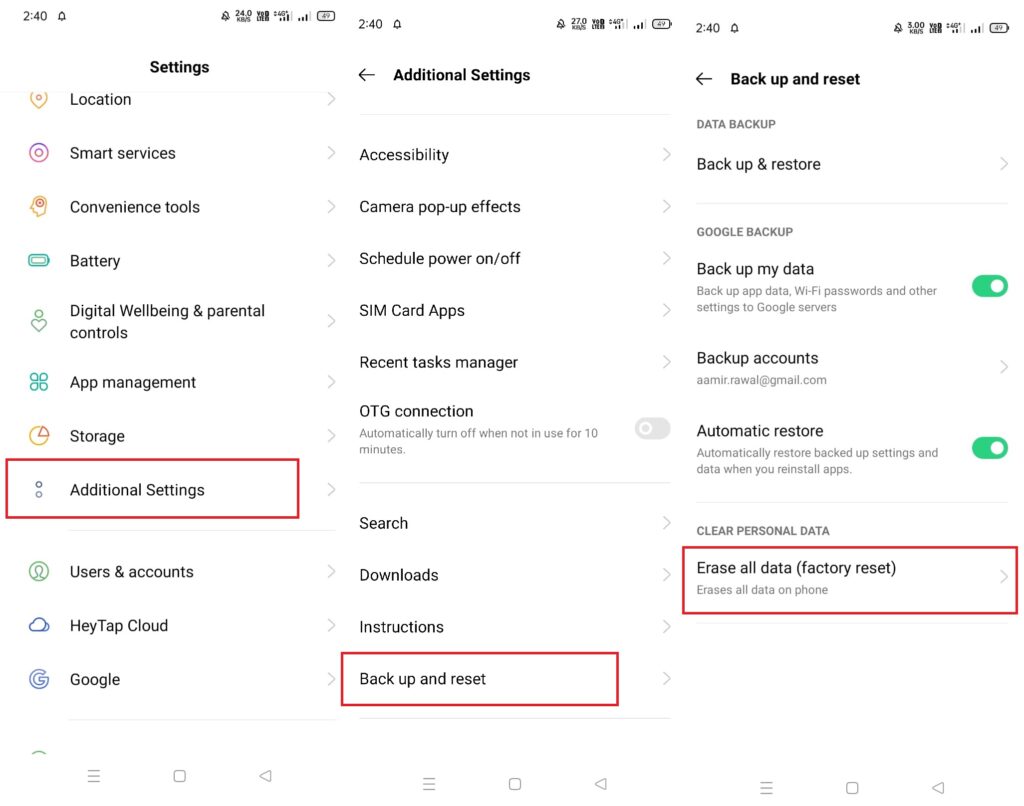The image depicts a detailed view of a multi-tiered settings menu, organized into three sections from left to right.

On the left, there is a primary menu on a white background labeled "Settings" in bold, black text. The menu lists several options:
1. Location
2. Smart Services
3. Convenience Tools
4. Battery
5. Digital Well-being & Parental Controls
6. App Management
7. Storage
8. Additional Settings, which is highlighted with a rectangular red border, indicating it is selected.
9. User and Accounts
10. Haytap Cloud (Note: 'Haytap' appears without a space)
11. Google

In the middle section, heading the menu, "Additional Settings" is prominently displayed in bold black letters with a left-pointing arrow beside it. The submenu options include:
1. Accessibility
2. Camera Pop-up Effects
3. Scheduled Power On/Off
4. SIM Card Apps
5. Recent Tasks Manager
6. OTG Connection
7. Search
8. Downloads
9. Instructions
10. Backup and Reset, which is also highlighted with a rectangular red border.

In the rightmost section, a focused view of the "Backup and Reset" menu is provided. At the top of this section, there is a left-pointing arrow beside "Backup and Reset". Below, in gray text, "Data Backup" is noted, followed by larger black text stating "Backup and Restore". Underneath, "Google Backup" is written in small gray font. The menu options here include:
1. Backup My Data (toggled on)
2. Backup Accounts
3. Automatic Restore (toggled on)
4. Erase All Data (Factory Reset), which is also highlighted with a rectangular red border, showing it is selected.

Overall, the image provides a comprehensive visual of the settings and backup options available, highlighting the specific sections and their current selections with red borders.